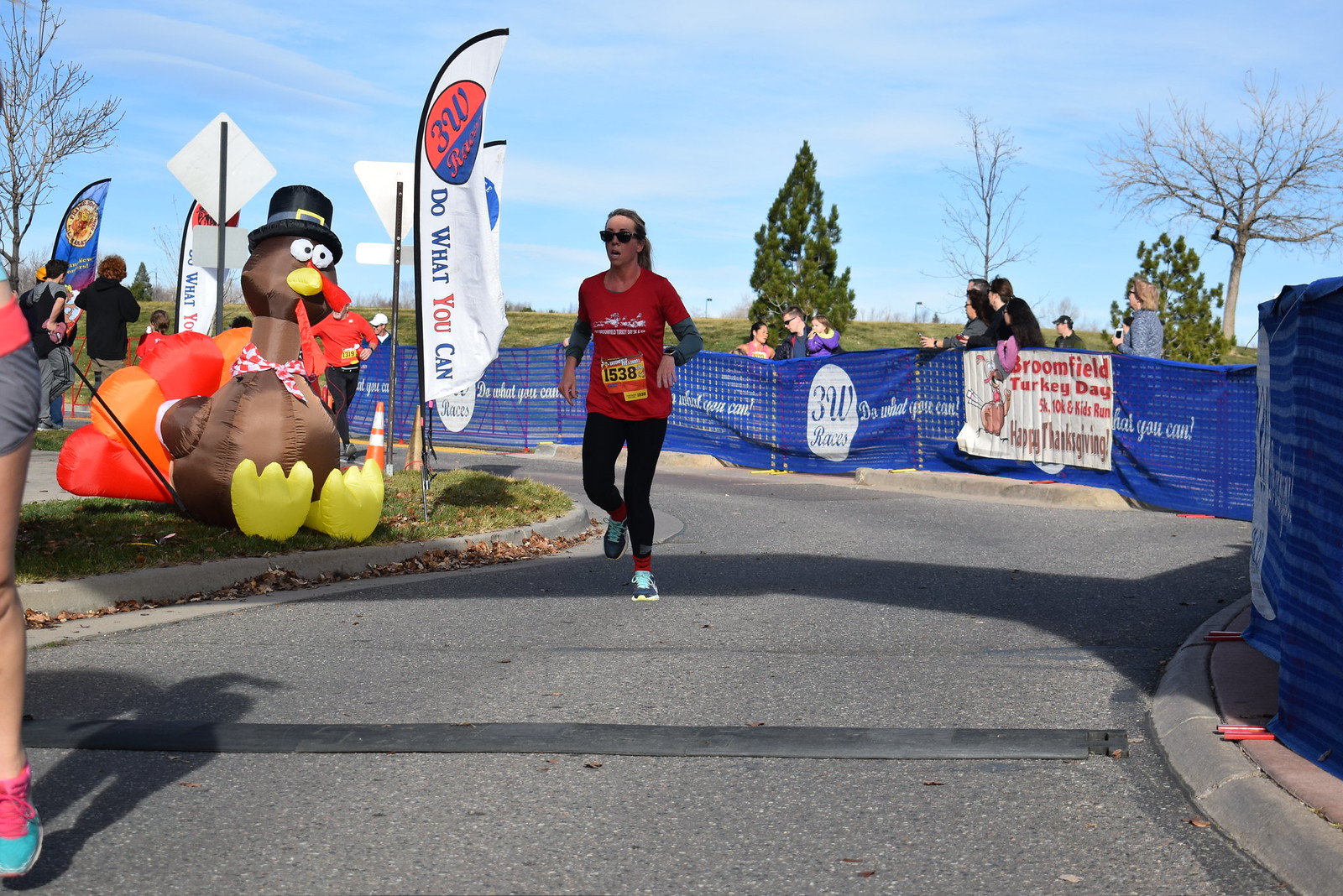In this vibrant full-color photograph capturing an outdoor daytime race, a female runner, wearing the number 1538, dominates the center of the image as she participates in a Thanksgiving-themed marathon. Flanking her on the left, an inflatable, stylized cartoon turkey adds a festive touch, indicating the holiday spirit of the event. The runner is on an asphalt single-lane road, which is bordered by a blue fence adorned with various advertisements and banners. Spectators, eager and engaged, line up behind these barriers to watch the race unfold. In the backdrop, a picturesque scene unfolds with a light blue sky and wispy white clouds overlooking a verdant field dotted with trees—some leafy and pointed, others barren with sprawling branches. Prominent banners and signs line the race path, displaying phrases like "Do What You Can," "3W Races," and "Broomfield Turkey Day 5K, 10K and Kids Run Happy Thanksgiving," highlighting both the charitable nature of the event and its various race categories. The overall composition blends lively colors—red, orange, yellow, green, blue, brown, and more—emphasizing the cheerful, community-focused atmosphere of this Thanksgiving marathon.